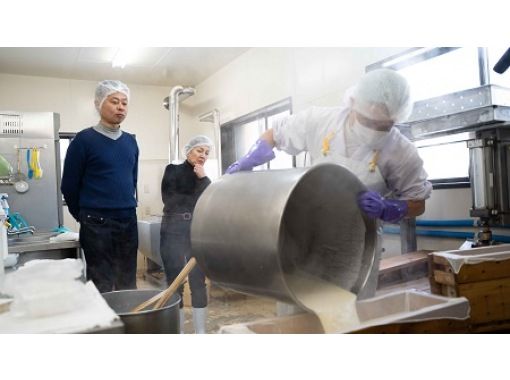In an industrial-style kitchen or food preparation area, three individuals are engaged in a meticulous process. The focal point is a man wearing heavy purple gloves as he carefully pours a cream-colored liquid from an oversized pot into a pan lined with cheesecloth. His actions are closely observed by two other individuals in the background, both dressed in white outfits complete with masks and hoods. Judging by the setup and the smooth texture of the liquid, it appears they are involved in the process of making cheese, possibly ricotta, as there are no chunks in the liquid.